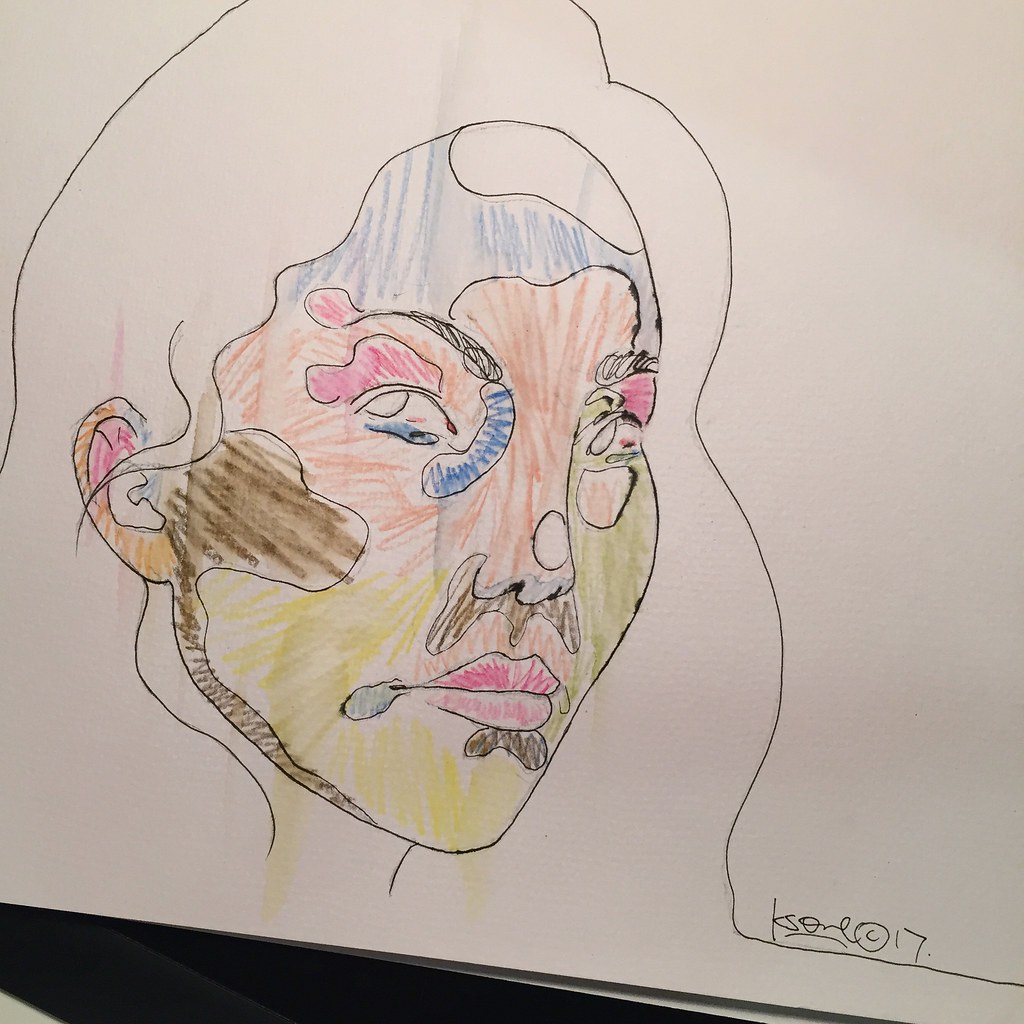The image depicts a detailed sketch of a woman's face, predominantly created using either pencil or black pen to establish the outline. This initial outline elegantly captures the contours of her long hair and facial features. However, the true highlight of the drawing is the face, which has been vividly colored with a mishmash of crayon or pencil hues in a chaotic, childlike manner. The colors diverge dramatically across different parts of the face: the left side of the face exhibits shades of brown, while the chin is covered in yellow, the right cheek turns green, and the forehead is awash in blue. Additional colorful elements include orange in the central area and red on her lips, with some pink and purple around her eyebrows. Each color segment almost resembles small facial tattoos, contributing an Asian-like aesthetic. Meanwhile, her hair remains uncolored, outlined in black and hinting at long, flowing locks that extend off the image. The right ear and some areas around the face display darker brown shades, possibly aiming to replicate shadowing effects. The image captures the face in a three-quarter view, allowing a focused study of the kaleidoscopic facial features. A curious detail is an indistinct artist's signature at the bottom right, paralleled by the number 17, with the bottom left corner of the sketchpad appearing black. This rich mix of colors and the intriguing execution imbue the drawing with a unique and dynamic visual appeal.